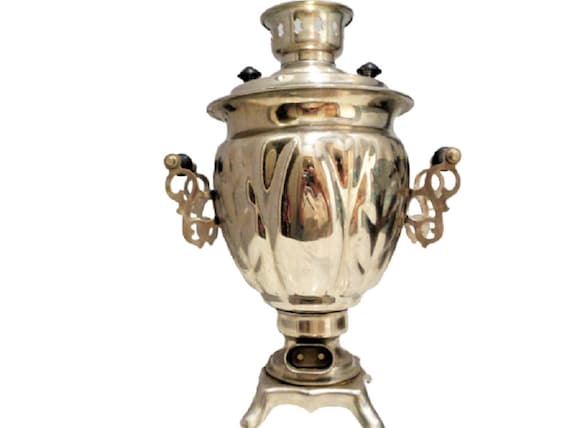This image showcases an intricately designed, antique-like metal urn or trophy, set against a stark white background. The object features a sturdy, roughly square base adorned with a fluted design and supported by four silver legs. Rising from the base, the urn’s neck is variegated and leads to a larger, more pronounced oval-shaped body. This main section is complemented by two elaborately crafted handles on either side, resembling ears in their creative design. The metal is highly reflective, showing hints of both silver and gold tones with visible reflections from the surrounding light and possibly the photographer. The lid of the urn is particularly detailed, with a small chalice-like structure on top, indicating a complex and functional design which might suggest usages such as a tea or coffee pot. The entire piece is meticulously assembled, indicated by visible black bolts and a seamless transition between various components.